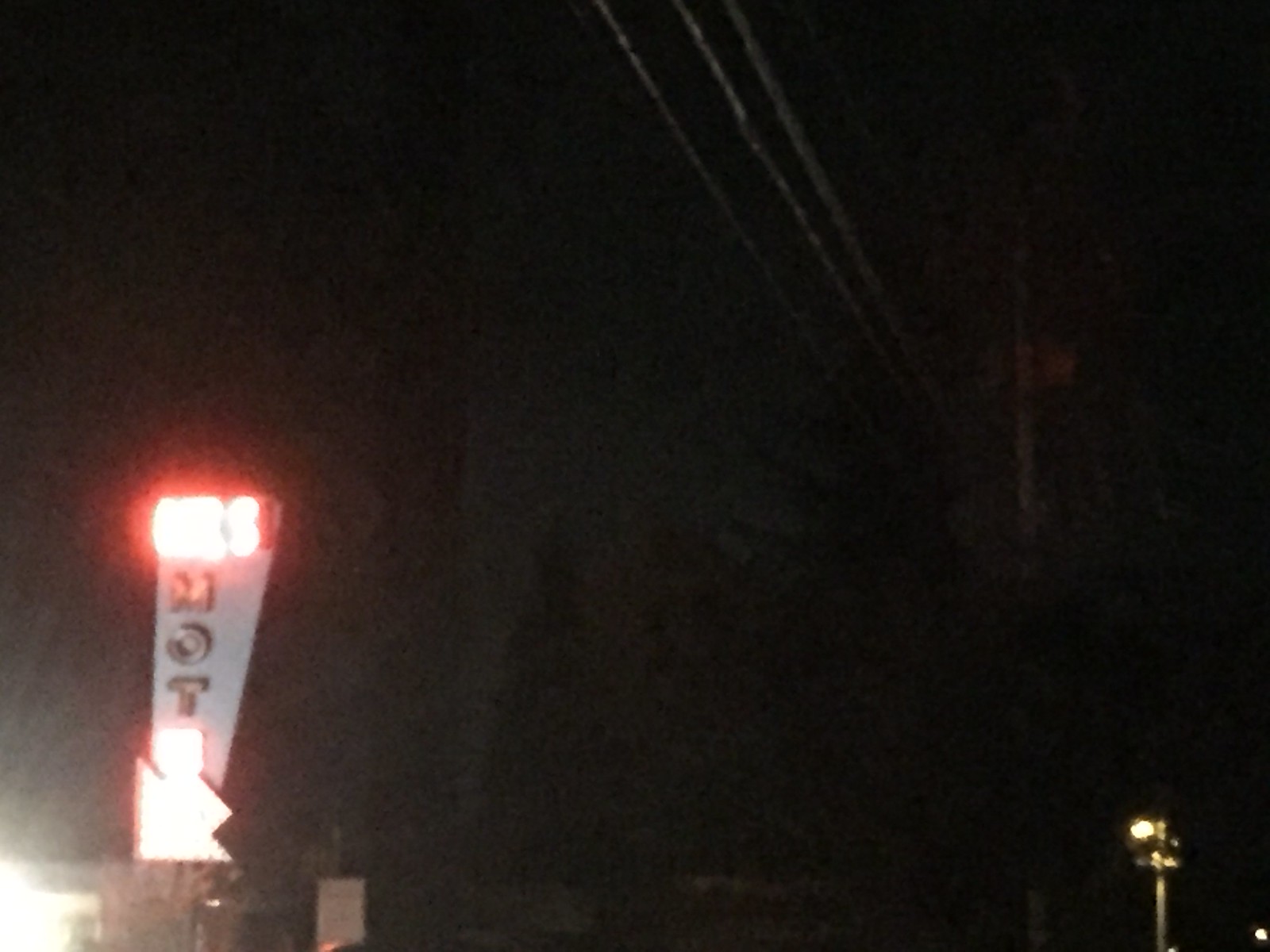A nighttime photograph taken from ground level captures a dark, almost pitch-black sky with minimal visible elements due to the low light conditions. In the left portion of the image, towering silhouettes of tall trees can be faintly discerned, adding to the eerie ambiance. The primary source of illumination comes from two light sources: a hotel sign and a traffic stoplight. The hotel sign, positioned vertically, features the word "HOTEL" and is designed in an abstract, asymmetrical shape resembling a triangle. Despite its brightness, the sign does not effectively illuminate any buildings, making the hotel itself indistinguishable. On the right side of the image, the stoplight adds a secondary glow, contributing just enough light to reveal a few power lines stretching across the scene above. The photograph's focus on upward angles emphasizes the power lines and obscures any additional ground-level details.